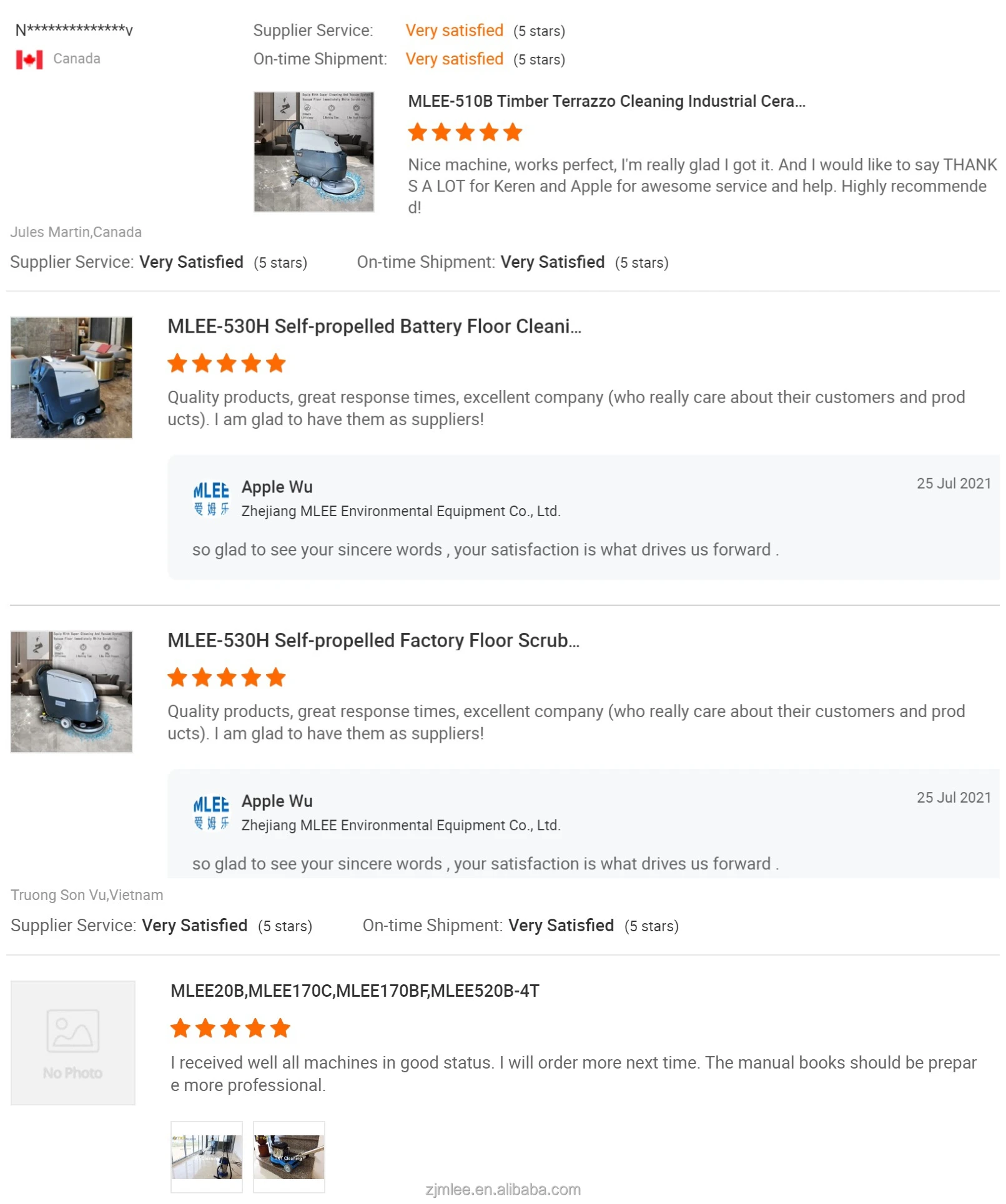This image showcases a section of a website dedicated to listing and reviewing various industrial cleaning products, accompanied by customer feedback and ratings.

At the top, the section highlights a supplier service, marked with a Canadian flag and the text "Canada." This signifies the region of service. The supplier service has received overwhelmingly positive feedback, boasting "very satisfied" ratings with five stars for both service and on-time shipment.

One prominently featured product review is for the MLE-510B Timber Terrazzo Cleaning Industrial machine, which has garnered a perfect rating of five out of five stars. The reviewer praises the machine as "nice" and "perfect," expressing immense satisfaction with their purchase and extending gratitude to "Karen and Apple" for their exceptional service and assistance, concluding with a strong recommendation.

Another detailed review comes from Jules Martin, also based in Canada. Jules reviews the MLE-530H Self-Propelled Battery Floor Cleaner, giving it five out of five stars. The review emphasizes the product's high quality, the company's excellent response times, and their customer-centric approach. Jules expresses contentment with having them as suppliers.

In response to Jules Martin’s review, the company, Apple Woo, gratefully acknowledges their customer's heartfelt words and expresses that customer satisfaction is their driving force.

Additionally, there is a consolidated review of multiple products, namely the MLE-202B, MLE-170C, MLE-170BF, and MLE-520B-4T, all receiving five-star ratings. The reviewer mentions that all machines were received in good condition and expresses intent to place more orders in the future. The commenter also suggests that the manuals could be more professionally prepared to enhance usability.

Overall, this image captures the essence of customer satisfaction and the quality of service provided by the supplier, showcasing detailed feedback and commendations for various industrial cleaning products.